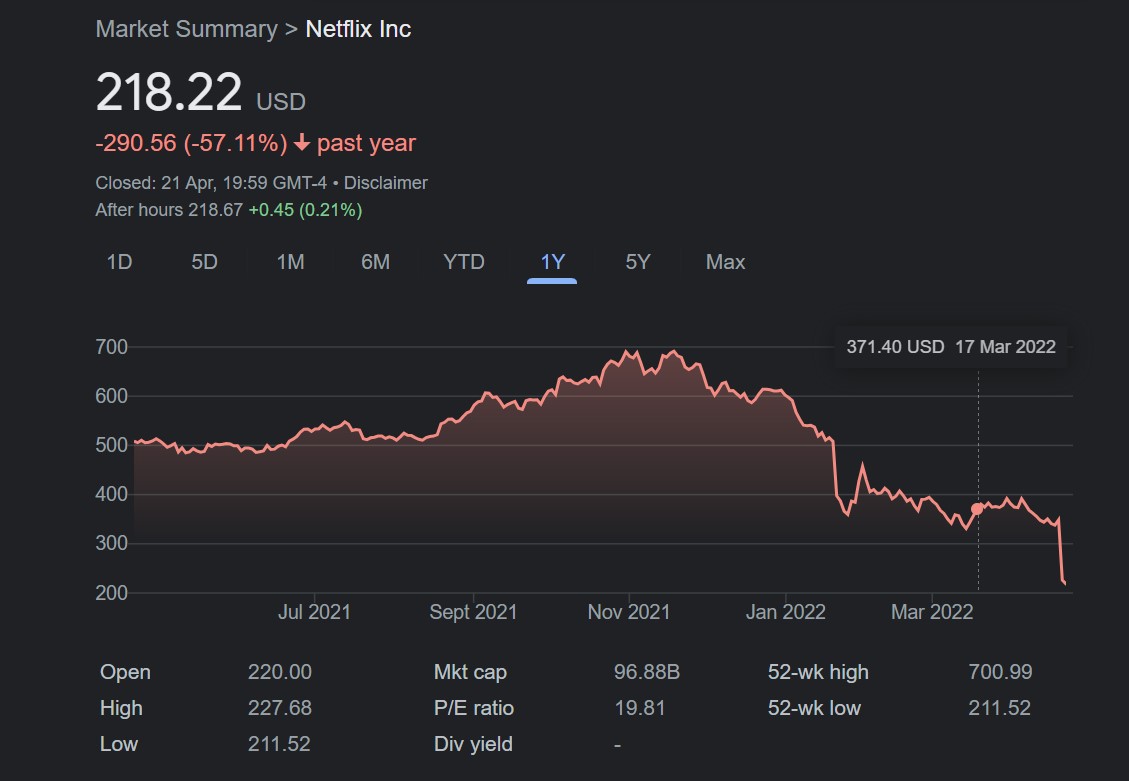This screen capture appears to be from a stock market summary for Netflix, Inc. The image is dominated by a large black background with text in varying colors—primarily white, but also red, green, and gray.

At the top, the header displays: "Market Summary Netflix, Inc." followed by a stock price of "$218.22 USD." Below this, in red text, it indicates a significant downturn with the details: "−290.56 (−57.11%)" over the past year, accompanied by a downward arrow. 

Further down, the text in gray states: "Closed 21 APR 1959 GMT−4." A disclaimer follows, showing the after-hours price in white text with green highlights: "$218.67 (0.45 or 0.21%)."

Continuing downward, the image shows several time-frame options in white and gray text: "1D, 5D, 1M, 6M, YTD, 1Y" with "1Y" highlighted in blue, indicating it is the selected option. Following this, there is a grey-colored text reading "5Y" and "Max."

A graph depicting Netflix’s stock performance is shown, with vertical markers at 200, 300, 400, 500, 600, and 700. The graph illustrates a peak close to 700 around July 2021. Timestamp markers indicate significant dates: September 2021, November 2021, and January 2022. The stock price begins declining sharply from January 2022 onward and remains low through March 2022, with an evident drop post-March.

Specific data points on the graph include: "371.40 USD, 17 March 2022." At the bottom, more details are displayed: "Open 222, High 227.68, Low 211.52," along with additional metrics: "Market Cap 96.88B, PE Ratio 19.81," and "Div Yield” is left blank. Notably, the 52-week high and low are listed as "$700.99" and "$211.52," respectively.